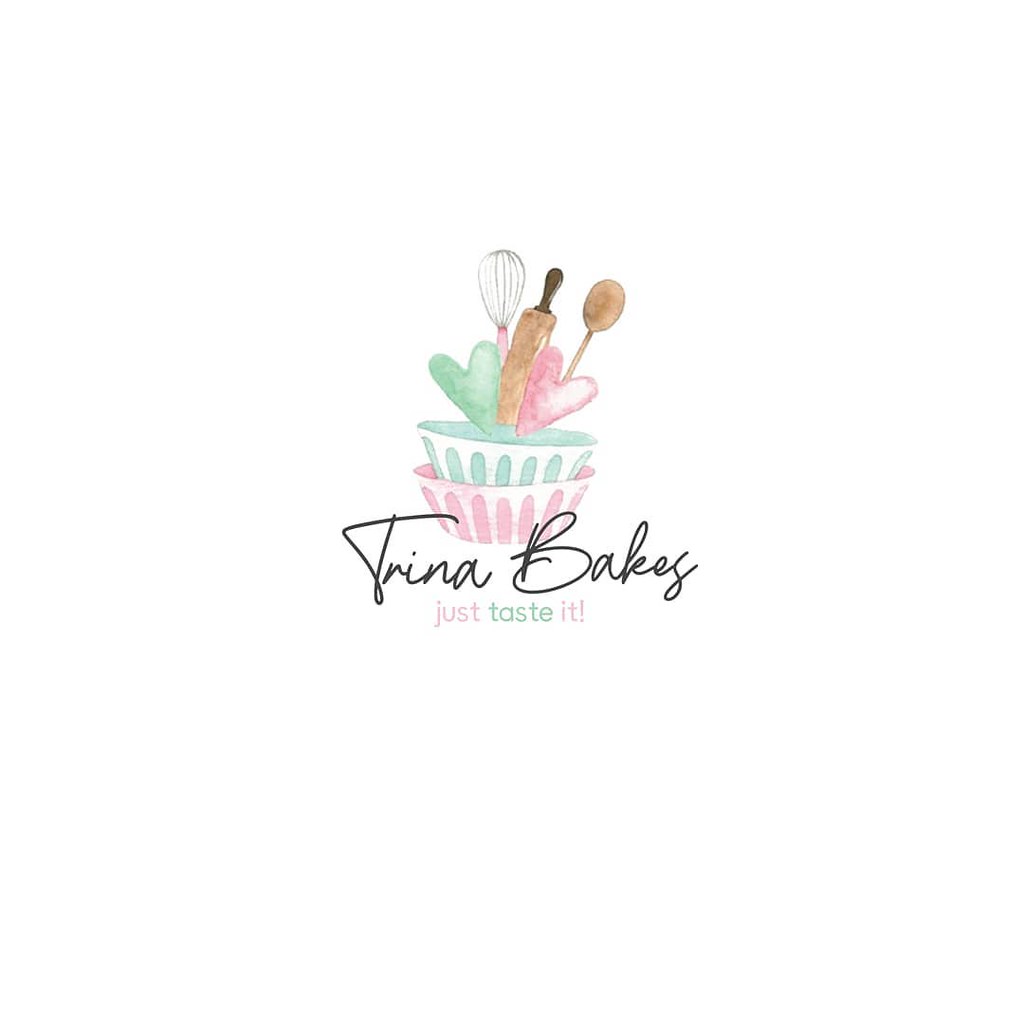The image is a detailed color illustration with a white, empty background, rendered in soft pastel colors with a watercolor effect. It features a stack of two nested baking bowls: the bottom bowl is pink, while the top bowl is light green. Inside the green bowl are several baking utensils – a beige rolling pin with dark brown handles, a wire whisk with a pink handle, and a wooden spoon. Among the utensils are two colored hearts, light green and light pink. At the bottom of the image, in cursive script, it reads "Trina Bakes," and below that, in a striking combination of pink, green, and orange typography, it says "Just Taste It!" This illustration merges graphic design and typography to likely serve as a logo or branding for Trina Bakes.